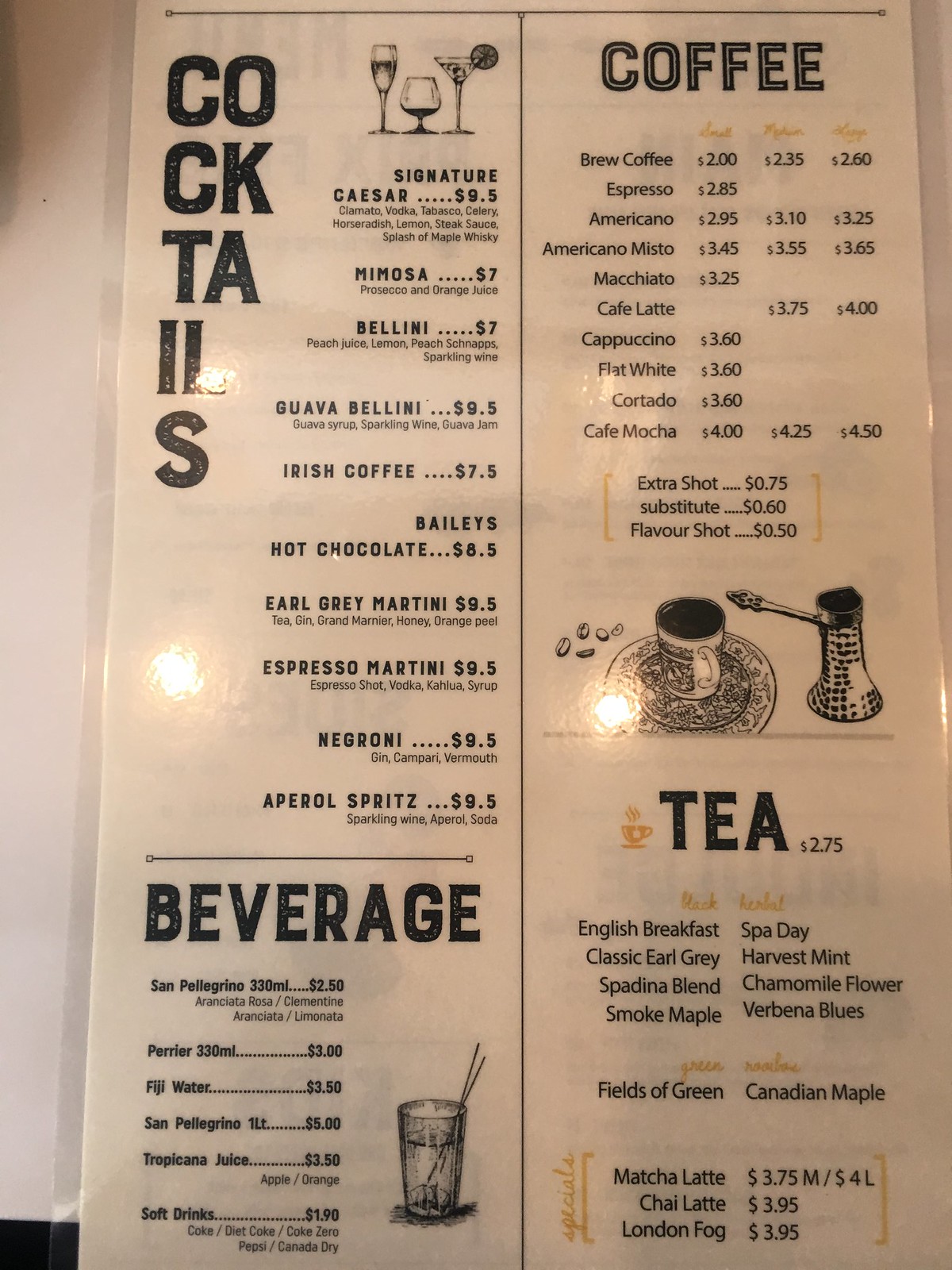This photograph features a laminated menu, evident from its glossy, easy-to-clean surface and the reflection of a flash, as well as background lights. Positioned against an off-white wall that complements its off-white background, the menu provides a detailed array of beverage options. In the upper right corner, there's an extensive list of coffees including brewed, espresso, Americano, and a variety of lattes and mochas. The lower right section is dedicated to a selection of teas such as English Breakfast, Classic Gray, Smoked Maple, and Harvest Mint. The lower left features an assortment of beverages like different kinds of water, juices, and soft drinks. The upper left corner highlights signature cocktails including Espresso, Hot Chocolate, Irish Coffee, Mimosa, and other exotic drinks. This menu suggests the establishment is primarily a beverage bar, focusing on coffee, cocktails, and tea, likely operated by a skilled barista.